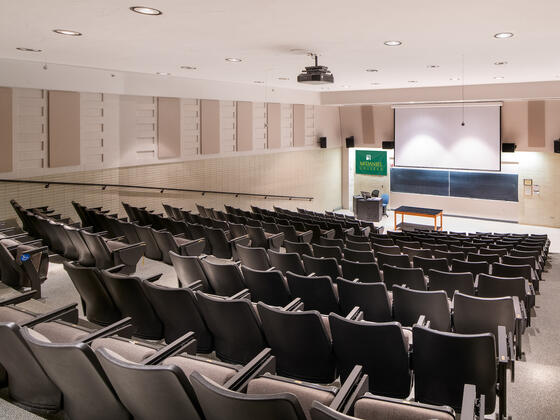The image depicts a college lecture hall with an auditorium-style layout. The room features eleven rows of chairs, split into two side sections with a central aisle. Each row has seven chairs and is arranged in a stepped formation, descending towards the front of the room where the professor's area is located. The professor's station includes a black rectangular wooden table with four legs, positioned centrally, and a personal desk to the left, equipped with a computer monitor and chair. Behind the professor's area, there's a double chalkboard and a large pull-down projection screen.

The walls and objects in the room exhibit a diverse palette of colors, including green, blue, orange, white, black, gray, tan, and beige. The ceiling is fitted with round recessed lights and a ceiling-mounted projector, aimed at the large screen. On the left side of the chalkboard, there is a stand, potentially holding a speaker or other equipment. The room is detailed with subtle features like the arrangement of the chairs and the various instructional tools, such as the banners and displays. Overall, the lecture hall is well-equipped for teaching presentations but is empty in this particular scene.